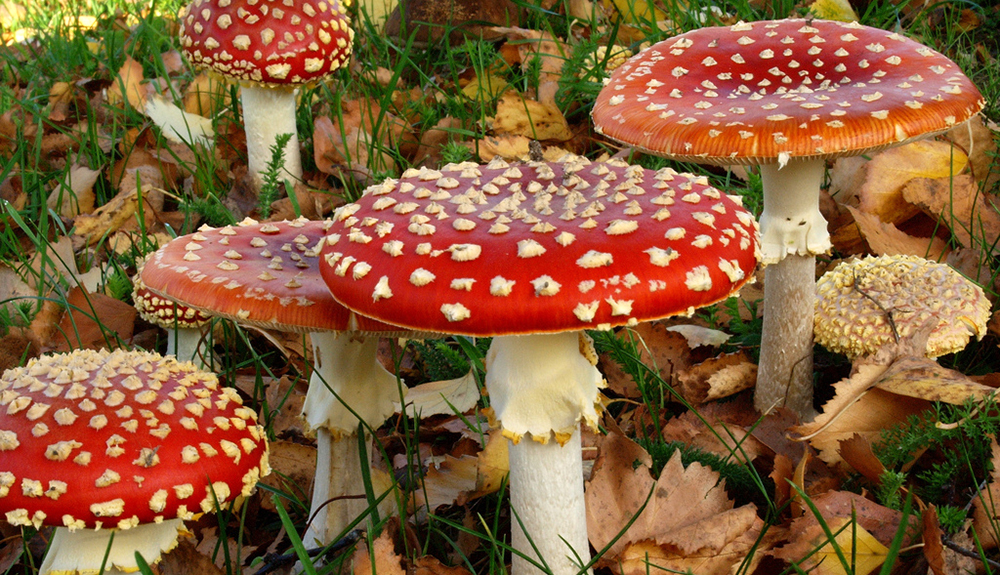This outdoor photograph captures a cluster of toadstool mushrooms set against a natural backdrop. Dominating the scene is a larger toadstool placed centrally, featuring a bright red cap adorned with distinct white splotches and supported by a white stalk. Arranged around it are four smaller mushrooms. To the left, three similarly red-capped mushrooms with white stems vary slightly in height and shape. The upper right corner showcases a somewhat orange-red toadstool, suggesting a different stage of growth or health, adjacent to a brown mushroom that contrasts with the otherwise vibrant group. The forest floor is scattered with brown, dried leaves mingled with green stalks of grass, echoing the earthy, autumnal setting. Sunlight filters onto some leaves in the top left corner, adding a touch of warmth to the scene. No text appears on this image, allowing the natural beauty of the mushrooms to take center stage.